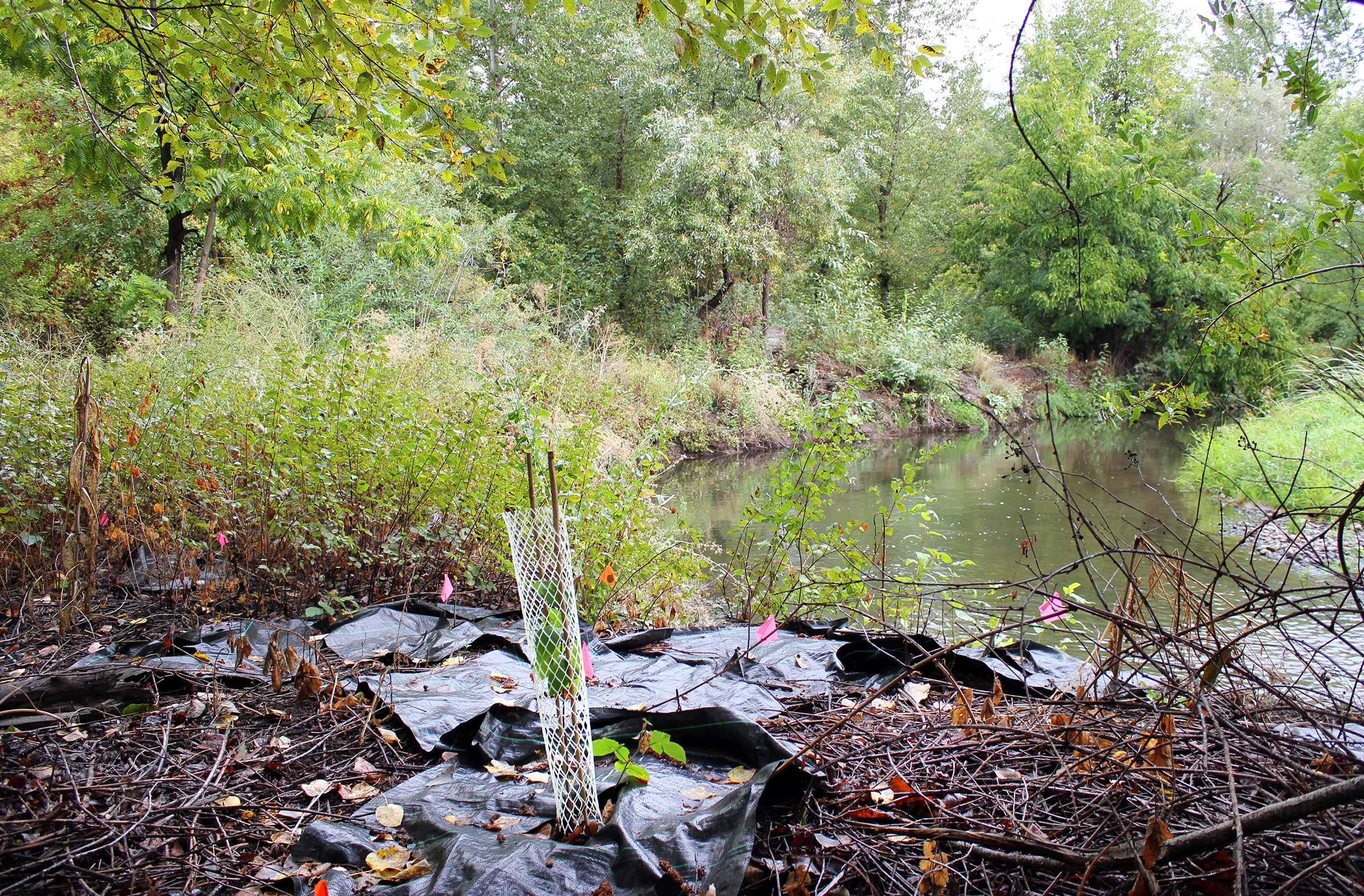In this outdoor photograph, a heavily wooded area envelops a marshy creek that winds from the right edge to the center and curves toward the lower right corner. The still water is flanked by a marshy edge and a grassy area filled with tall, reedy grass and shrubs, leading up to tall, verdant trees in the background, with only a slight sliver of sky peeking through the upper right. The foreground features a mixture of muddy or gravelly terrain with gray rocks and brown twigs scattered about. Prominently displayed in the center or slightly to the right is a black tarp, partially covering fallen brown tree branches. Sitting atop the tarp is a white mesh wire cylinder, about two feet high, supported by two brown posts. Inside this cylinder, a young sapling with green leaves is growing, seemingly nurtured for new growth amidst the dense surrounding forest. Additionally, small pink flags are attached to the area, marking it as a site for ongoing or planned planting, possibly to introduce native plants. A few low-lying trees and brambles without leaves add to the diverse layers of foliage in this serene, forested scene.